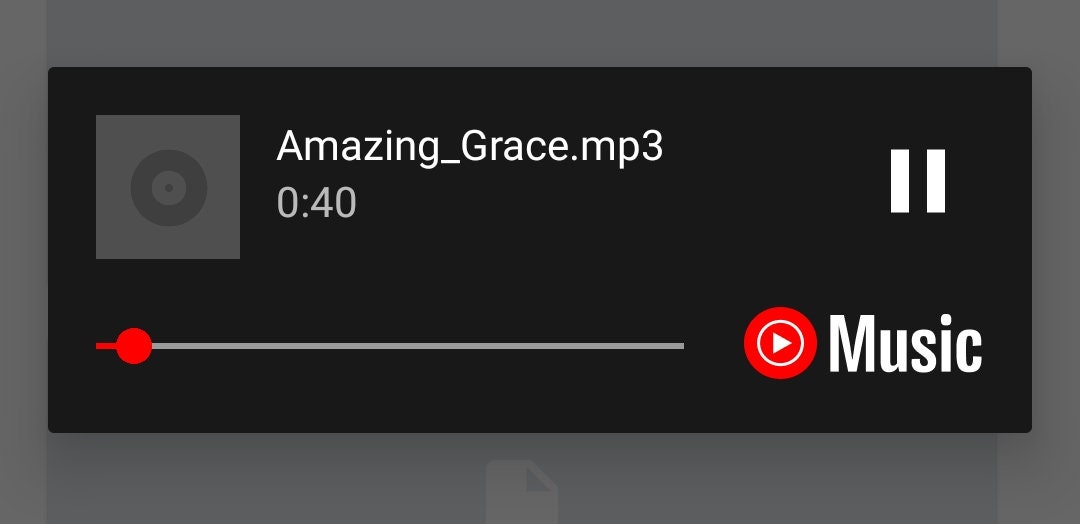A detailed descriptive caption for the image might read:

"This landscape-oriented screenshot showcases an abstract grey background, with varying shades creating an in-and-out pattern effect. Prominently featured in the center is a black rectangular area, indicating the main focus of the screenshot. 

In the bottom left corner of this black section, there's an almost stationary slider with a barely moved red button. To its right, a red circle with a play button icon sits beside the word 'music' in white text, suggesting that this is a media player, likely YouTube Music.

The upper left corner of the black section includes a grey square with a central circle next to the filename 'amazinggrace.mp3', providing context for the playing audio. Beneath this, the timestamp reads '0:40 seconds,' showing the current point in the audio track. Dominating the upper right corner of the black section is a large, easily accessible pause button, indicating the audio is currently playing.

Additionally, a small white icon or design is visible in the bottom center, adding a subtle accent to the otherwise minimalist display. The overall composition suggests that the media player is actively playing 'Amazing Grace', having progressed about 1% through the track with an option to pause available."